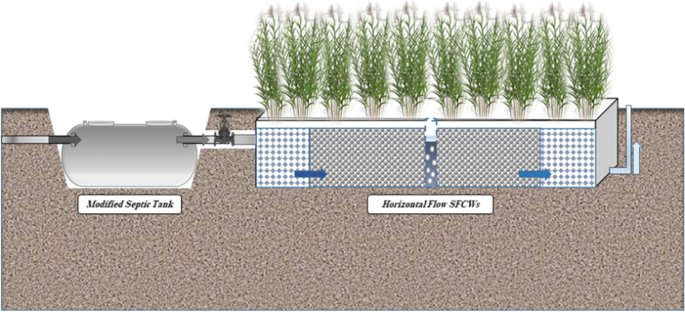The image is a detailed illustrative drawing, likely intended for use by contractors or engineers, depicting an underground modified septic tank system integrated with a horizontal flow Subsurface Constructed Wetland (SFCW). The in-ground septic tank, shown in gray, features a series of pipes and a valve, directing water and residue into the SFCW setup. This setup resembles a greenhouse or nursery, housing approximately 10 green plants with beige stems arranged in a row at the top. These plants are nourished and irrigated by the wastewater and nutrients from the septic tank. Additionally, a vent pipe is visible, extending up to the surface. Text annotations on the image label various components, including the modified septic tank and the horizontal flow SFCW.